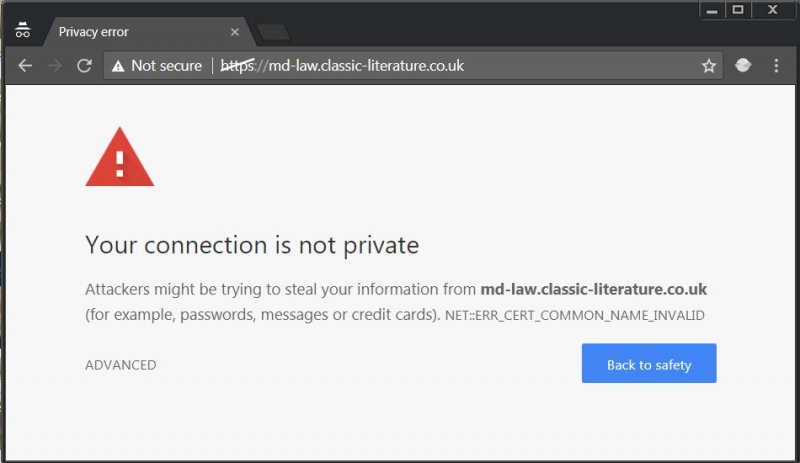The top section of the website features a black background on the left-hand side, suggesting that the user is browsing in incognito mode. A white hat and glasses icon reinforce this notion. The browser tab displays a gray background with the text "Privacy error" in white, accompanied by a small "X."

The top toolbar has a white line, including a white-outlined box with an "X" inside it, a white left-pointing arrow, and a gray right-pointing arrow. Next to these icons is a gray search box containing a white triangle with a black exclamation point. The text within the search box reads "Not secure," indicating a potential issue with the website's security. The URL "https://md-lore.classic-literature.co.uk" appears crossed out in white.

Moving to the actual webpage content, which is light gray, there is a prominent red triangle with a white exclamation point in the center. Below this symbol, the warning message "Your connection is not private" is displayed in black text. Further details explain that attackers might be trying to steal information from "md-lore.classic-literature.co.uk," including passwords, messages, or credit card details. The error code "NET::ERR_CERT_COMMON_NAME_INVALID" is also present, followed by options labeled "Advanced" and "Back to safety" in white text. The upper section of the page features three vertical white dots on the right side, denoting a menu or additional options.